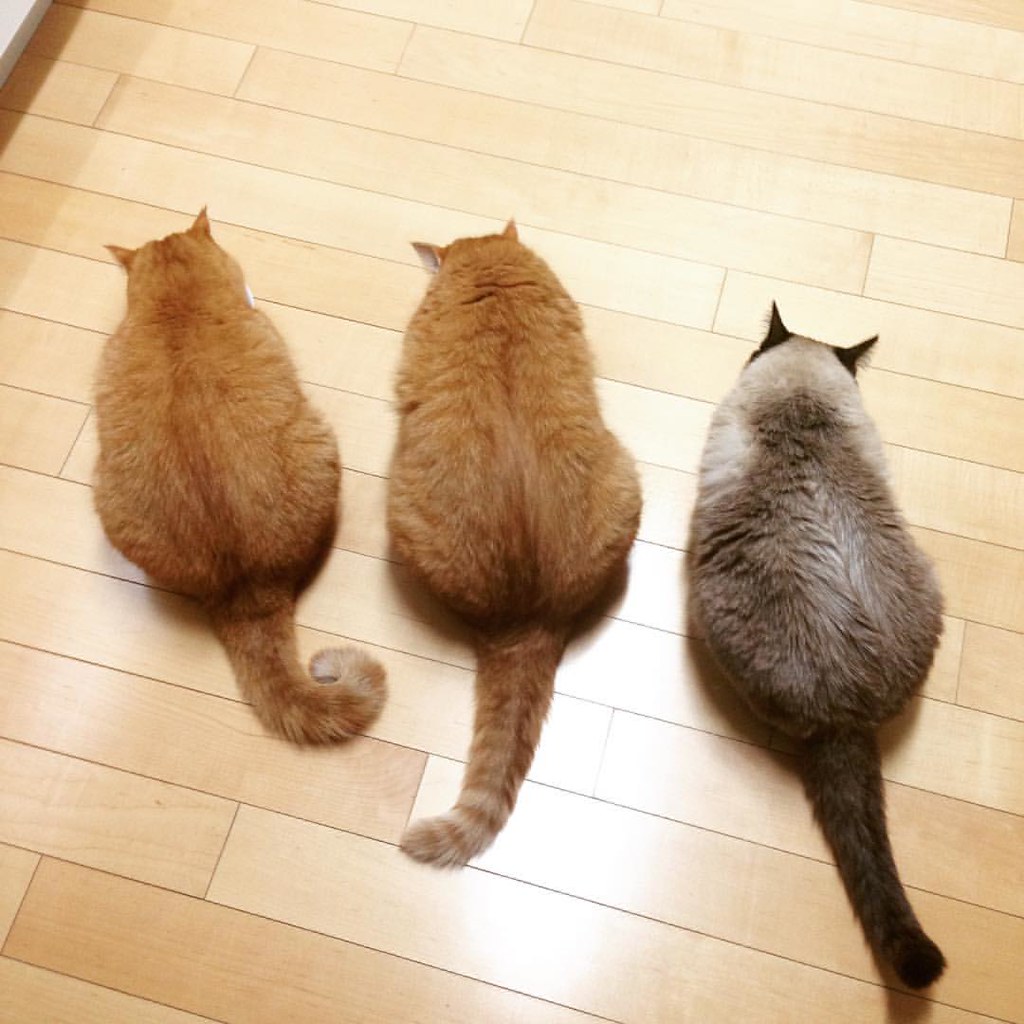In this photograph, we see three cats laying side by side on a light-colored, white, wooden tiled kitchen floor, viewed from above. The two cats on the left are orange with the one on the far left having a curled tail and the one in the middle having a straight tail with a striped pattern alternating between white and ginger. The cat on the right is a mix of brown and white, with distinctive black ears, and a black tail extending out of the frame. All three cats are facing away from the camera, presenting a serene and uniform arrangement on the light blonde, possibly maple, flooring.